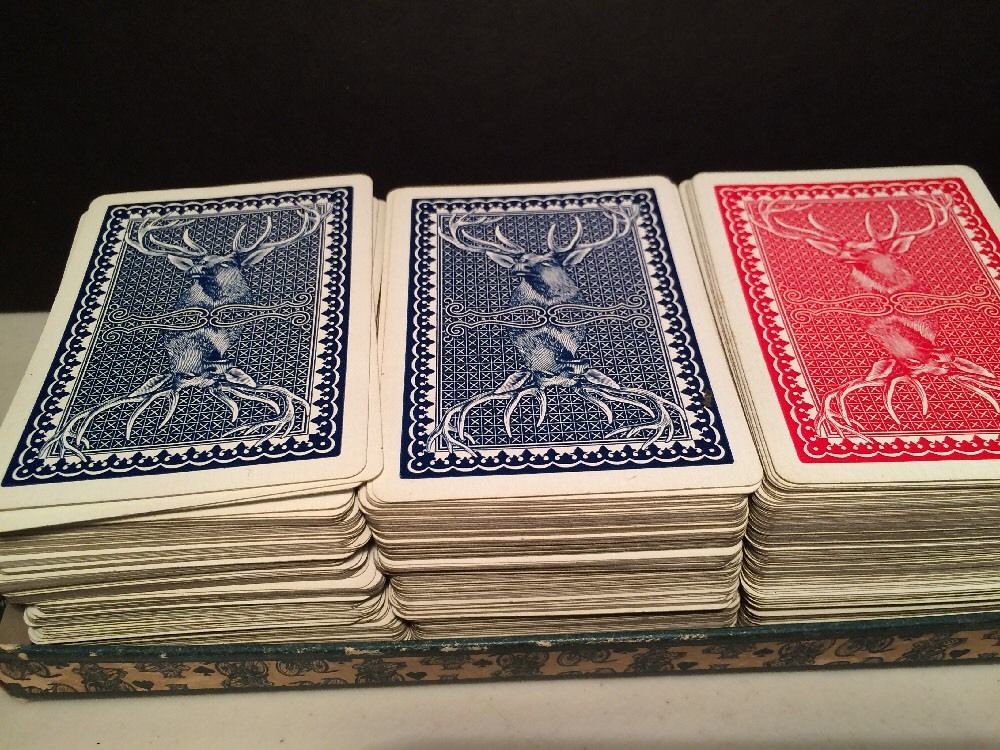The image showcases three old decks of playing cards arranged side by side. The decks are visibly aged, with significantly yellowed borders. The red deck sits between two blue decks, each displaying various levels of aging and discoloration. One blue deck is a darker shade, while the other is a lighter blue, both featuring equally yellowed white borders. 

The cards in the red and darker blue decks are neatly stacked, while the lighter blue deck on the left is slightly disheveled, with a few cards leaning towards the middle stack and a general unevenness throughout the pile. 

All three decks rest on a two-toned stand, predominantly green with worn, tan edges where the green has faded away. The stand itself is placed on an off-white table against a stark black background. The worn condition of both the cards and the stand adds a layer of vintage charm to the composition.